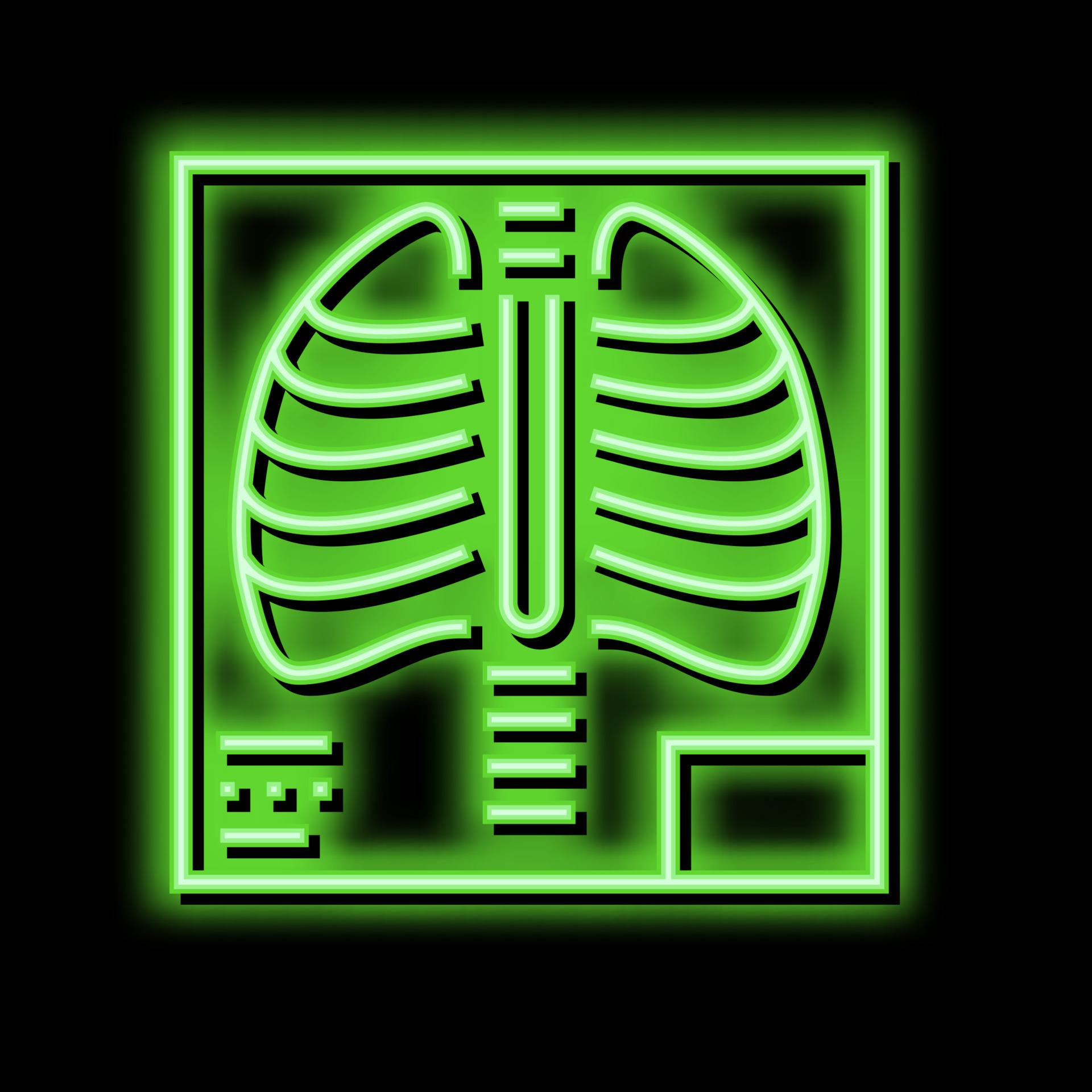The image features a solid black background with a neon green square prominently displayed in the center. Inside this square, there is a detailed graphic that bears a resemblance to a human ribcage and spinal column. The spine is depicted as a series of green rectangles stacked vertically, with four at the bottom and two at the top, while the ribcage is formed by curved horizontal lines on either side of the spine. The center of the square is so brightly illuminated that it nearly appears white, emphasizing the fluorescent green hues around it. Additionally, the lower left corner of the square contains a symbol composed of two horizontal lines with three small dots in between, and the lower right corner features a straight line that nearly forms a rectangle. The entire neon graphic has the appearance of a lit-up neon sign, with its vivid green lines standing out starkly against the black background.